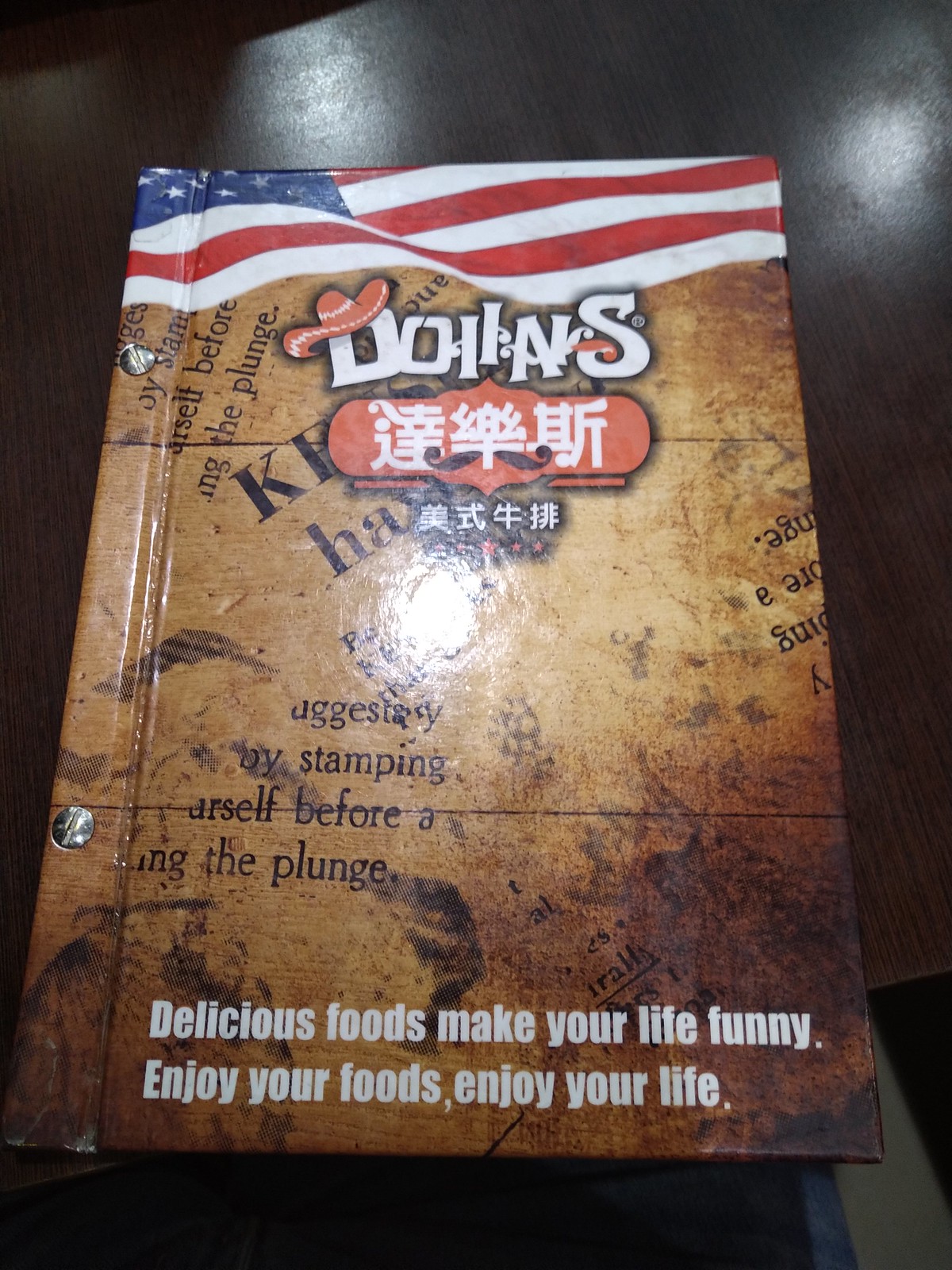The image captures a hardcover book placed on a brown table. The book cover features an American flag at the top. Beneath the flag, there is an unfamiliar word, which appears to be "D-O-I-I-A-I-S", followed by Japanese or Chinese characters. The background of the cover is predominantly brown with scattered, random words. Among them, a partially stamped message reads, "SUGGEST BY STAMPING YOURSELF BEFORE THE PLUNGE". Near the bottom of the cover, white text reads, "DELICIOUS FOODS MAKE YOUR LIFE FUNNY, ENJOY YOUR FOODS, ENJOY YOUR LIFE". The book is secured with two screws or bolts in the middle region.